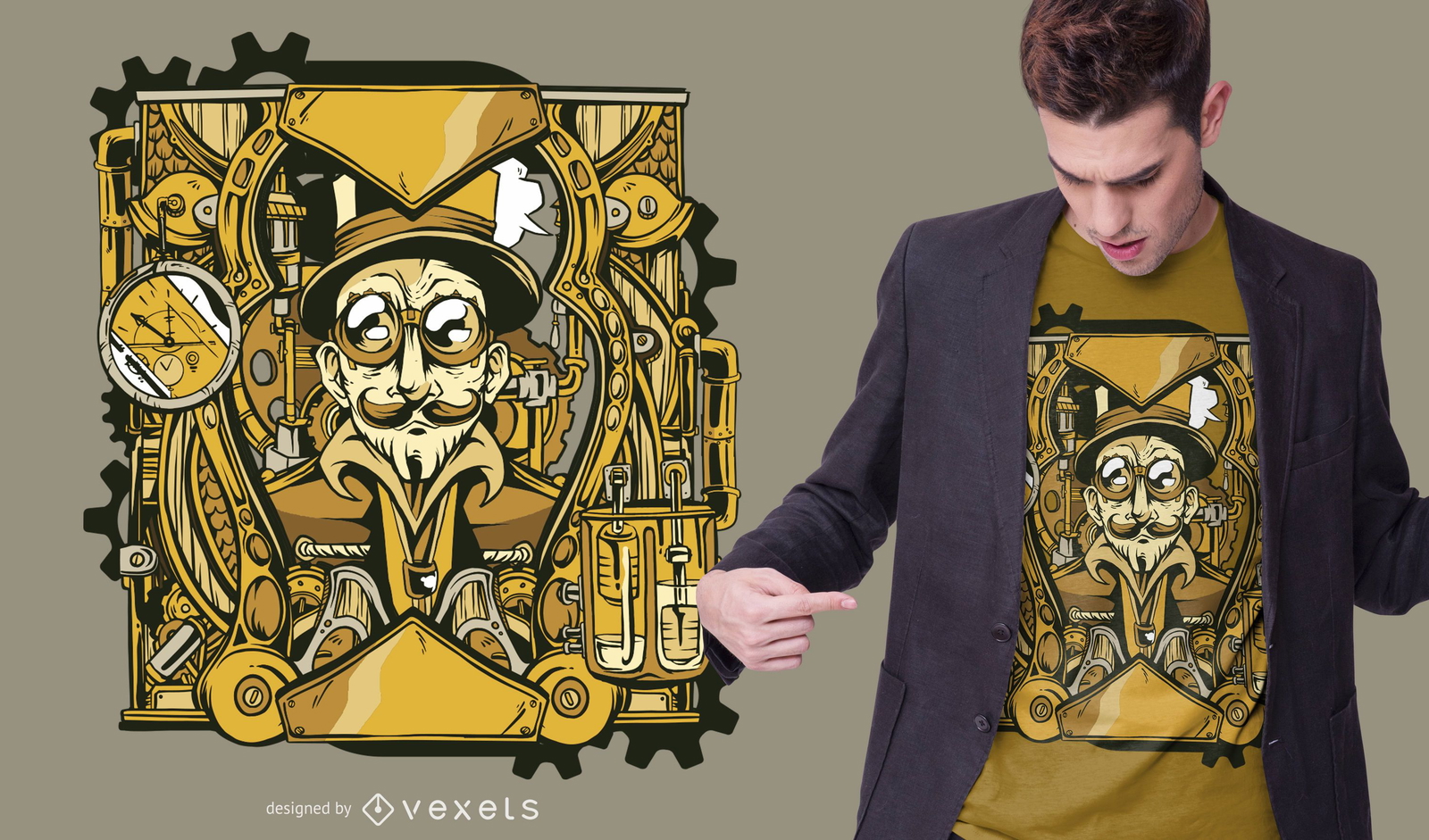The image is a detailed advertisement featuring a clean-shaven man with brown hair, dressed in a black open vest jacket over a golden shirt with an intricate steampunk design. The man, positioned on the right side of the image, is looking down and pointing at the design on his shirt. The golden shirt features a stylized steampunk man with an upward-curling handlebar mustache, big goggles, and a top hat, all rendered in various shades of gold and black. The steampunk figure is surrounded by gears, pipes, and other intricate machinery. Below this design, which is primarily colored in golds and blacks, the text reads "Designed by Vexels," with a small diamond-shaped logo between the words. On the left side of the image, a close-up view of the steampunk design is shown against a solid earthy green background, highlighting the detailed artwork on the shirt.